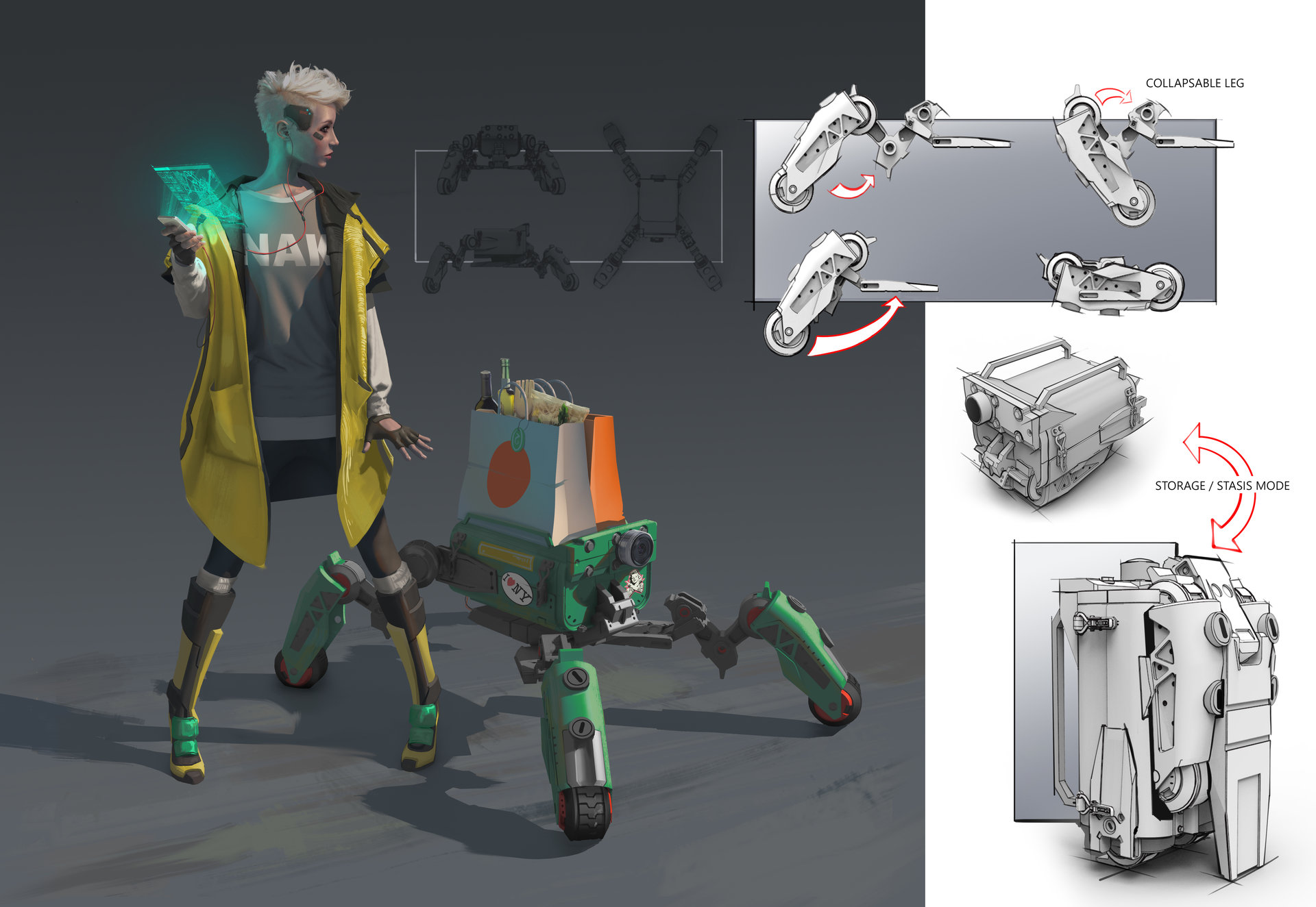The image portrays a detailed animation scene set against a black background, featuring a futuristic woman and her robotic companion. The woman, sporting short white hair, appears on the left side. She is dressed in a distinctive outfit that includes a gray and white long-sleeved sweatshirt underneath an oversized yellow and black jacket with visible pockets. She pairs this with black leggings, knee-high black fingerless gloves, and striking gray, yellow, and green knee-high boots. Attached to the right side of her temple is a computer chip with wires trailing around her ear, suggesting a digital or cybernetic enhancement. Illuminating her right hand is a neon green screen, potentially a holographic or 3D display emanating from a device she holds.

Beside her stands a small green, four-legged robot equipped with wheels and laden with an orange and a white shopping bag; the latter bag appears to feature an orange graphic. This robot serves as her practical helper, designed to carry her groceries. Adjacent to the robot are detailed illustrations in black and white, labeling features such as "collapsible leg" and "storage stasis mode," indicating the robot's ability to fold and compact itself when not in use. Additionally, there is a diagram of what looks to be a pocket knife among the futuristic metallic devices depicted. This comprehensive scene epitomizes an advanced, cyber-infused daily life.